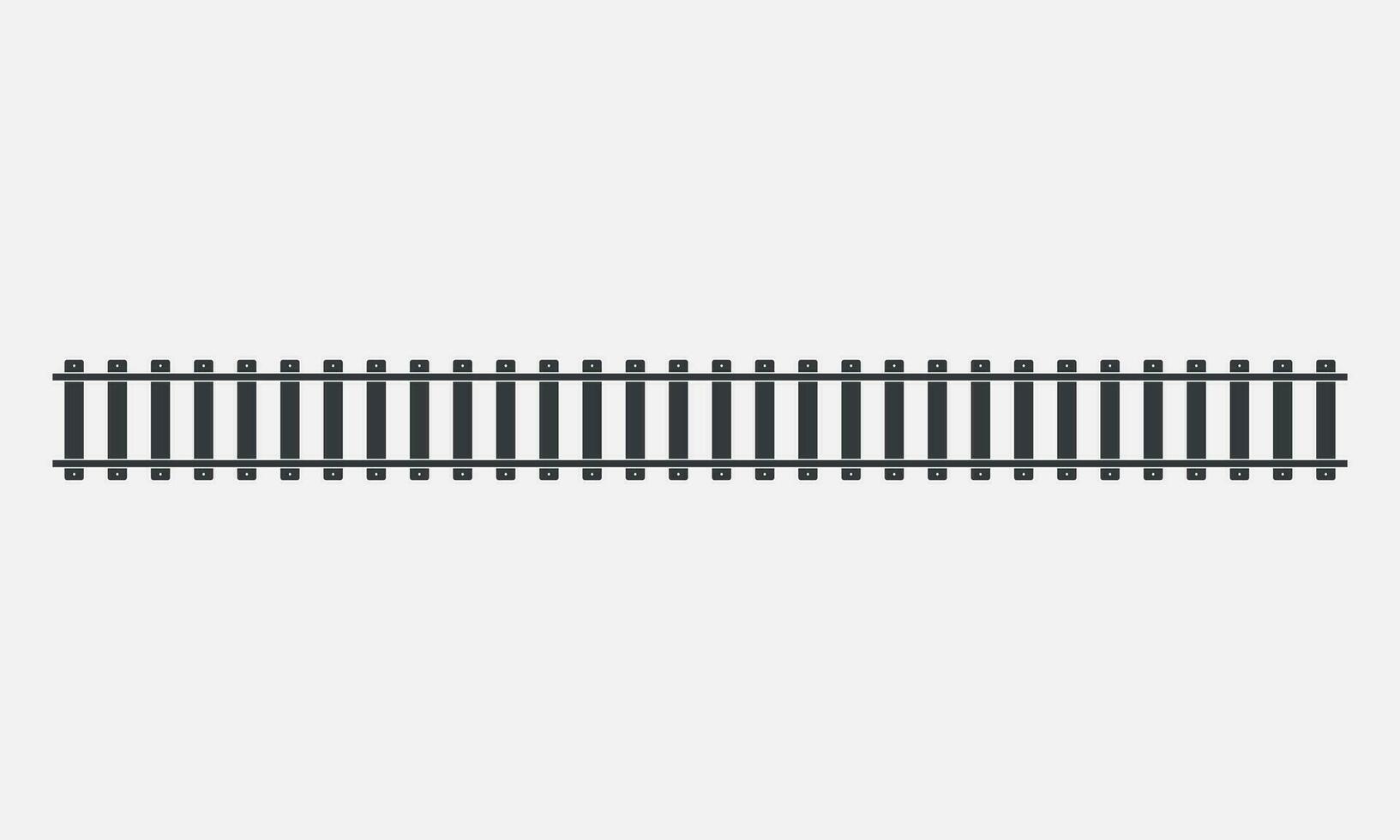The image features a minimalist illustration placed centrally against a very light, nearly white background. At the center is a structure resembling a railroad track. The track consists of two long, horizontal, dark gray rails extending from the left center to the far right center of the picture. Between these rails are vertical black planks or slats that resemble either the crossbeams of a railroad track or the boards of a black wooden picket fence. The planks do not fully reach the edges of the image, leaving small gaps at both ends. Little white dots, possibly representing railroad spikes, are visible at regular intervals where the rails overlap the planks. The entire composition creates an effect that can be interpreted either as a segment of a railroad track or a stylized fence, set against the light background.